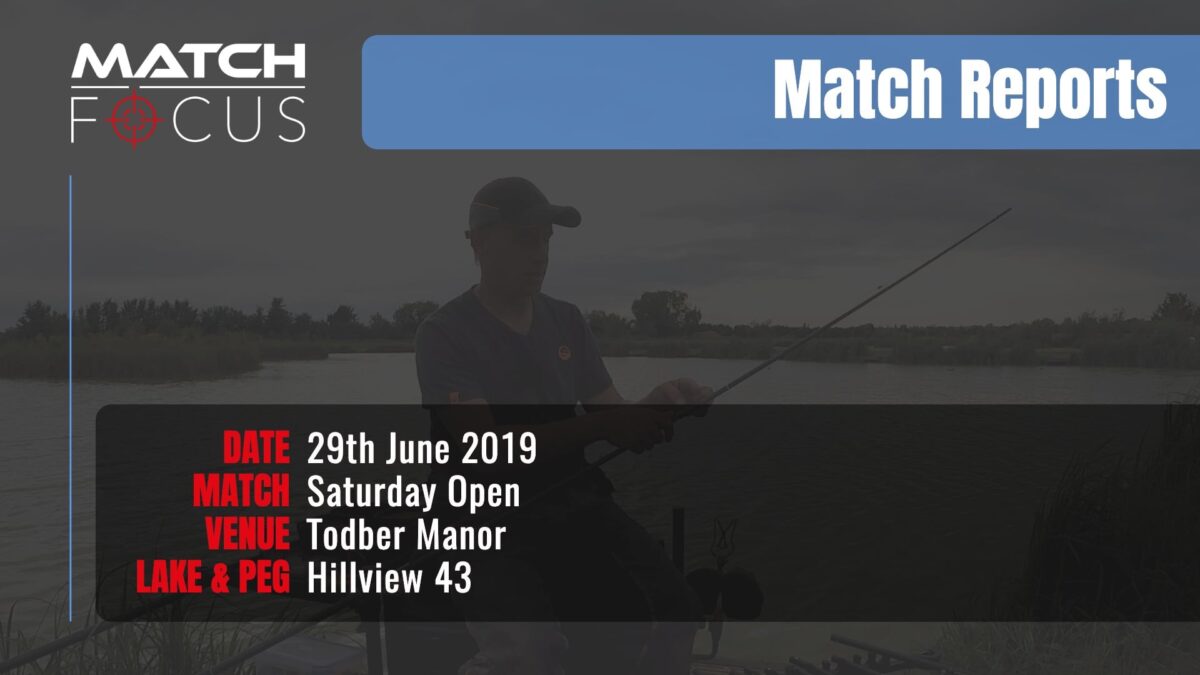The image is a poster advertising a fishing competition. The dark background features a central figure of a man, who appears to be fishing from either a boat or a dock. He is holding a fishing rod, wearing a baseball cap, and casting a line over a body of water. The scene includes a tree line and a sky in the distance, suggesting an outdoor setting in the middle of the day. 

In the upper left corner, "Match Focus" is displayed, where the "O" is a red bullseye. To the right, a blue band with rounded corners contains the white text "Match Reports." At the bottom, a larger dark rectangle runs almost the entire width of the image, with varied text details: "Date: 29th June 2019" in red and white, "Match: Saturday Open", "Venue: Todber Manor", and "Lake and Peg: Hill View 43." The colors predominantly used are blue, white, gray, black, and red, with different shades of gray.